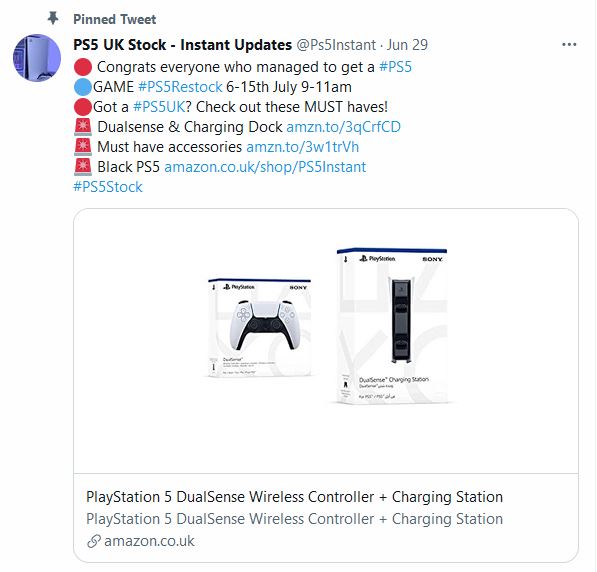This is a cropped screenshot of a social media post featuring a white background. In the top left corner, there is a dark gray pushpin icon, next to which appears the phrase "Pinned Tweet" in dark gray text. Below this, on the left, is a circular profile picture displaying a vertically oriented white gaming console with a purple-lit background. 

To the right of the profile picture is the username "PS5 UK Stock Dash Instant Updates" in bold black text, followed by the handle "@PS5Instant" and the date "June 29" in light gray text. Further to the right, aligned to the far end, are three dark gray horizontal dots.

Beneath the username, various icons and text lines are arranged. The first row starts with a red dot followed by the message, "Congrats everyone who managed to get a," with the term "#PS5" in blue. The next entry features a blue dot with the message in all caps, "GAME #PS5 Restock," followed by the dates "6 to 15th July" and the time "9 to 11 a.m." in black. 

The next line starts with a red dot reading, "Got a #PS5UK? Check out these MUST-HAVES," with "MUST" emphasized in all caps. Then, three red emergency light icons list recommended accessories. The first one states "DualSense and Charging Dock" with a link: "AMZN.TO/3QC RFC D" in blue. The second suggestion reads "Must-have Accessories" accompanying another link: "AMZN.TO/3W1 TRV H" in blue.